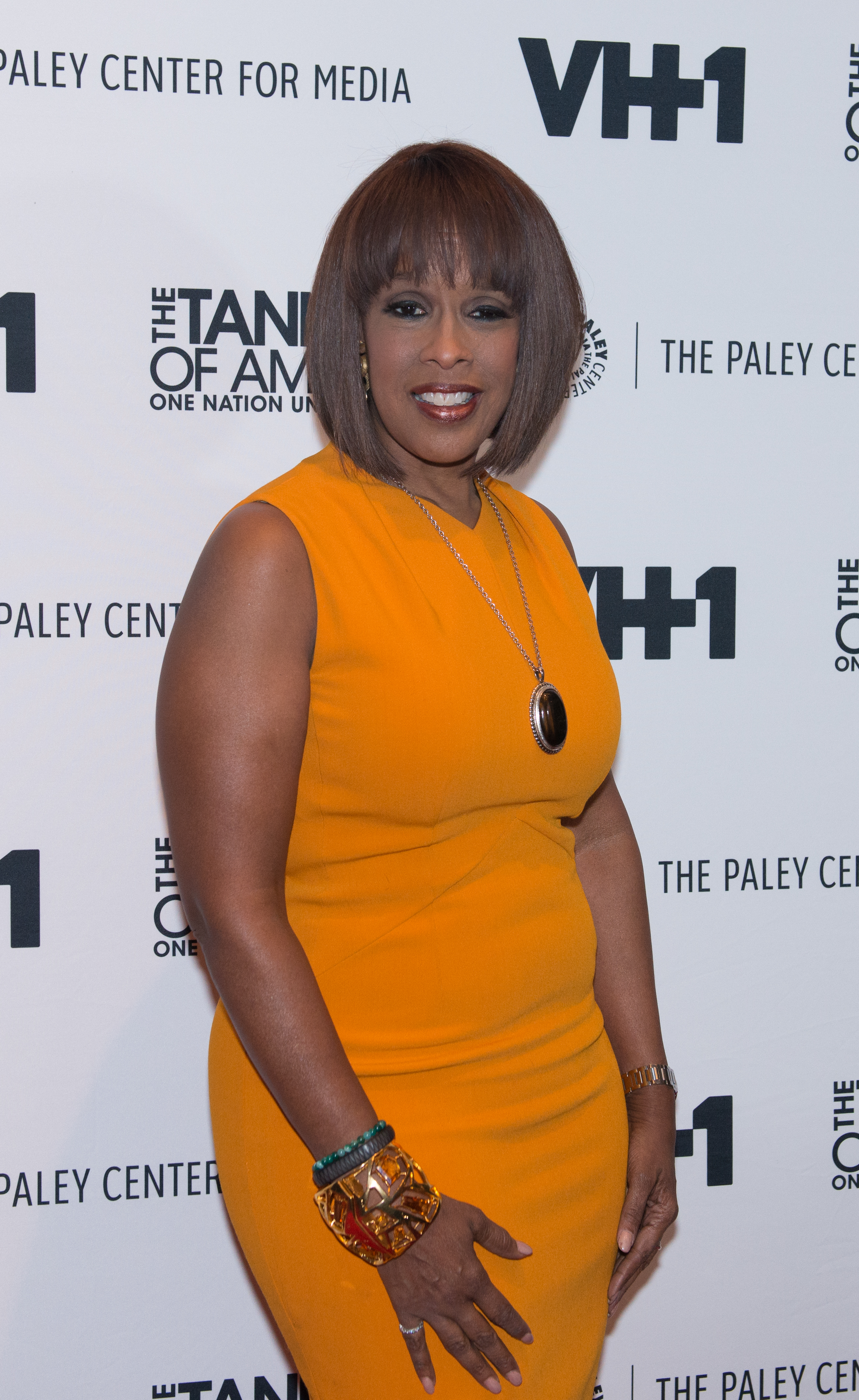In the photograph, there's a close-up of an African-American woman, likely a celebrity, posing confidently in front of a branded white wall backdrop. The backdrop features logos and text, including the Paley Center for Media and VH1, with parts of other words partially obscured by her head. She has medium-length brownish-black hair that reaches her neck and shoulders, and she is adorned with dark red or light reddish lipstick, and noticeable eye shadow. She is wearing a striking, sleeveless, form-fitting dress in an orange-yellow hue. Around her neck, she has a prominent metal locket pendant with a black centerpiece. On her right arm, she sports several bracelets, including a large, see-through one with shades of orange, yellow, and red, along with some blue ones, and a gold-toned wristband or bracelet. There is also a visible bracelet or watch on her left hand. The woman is smiling brightly, showing all her top teeth, and her right eye appears slightly smaller than her left.